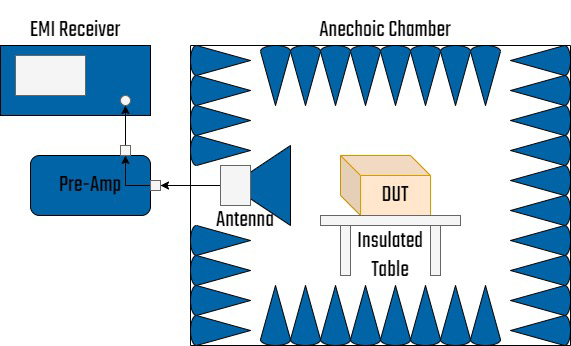The image depicts a detailed schematic or flowchart for an electrical device or system. The main section of the image is dominated by a large white rectangle with a black border, inside of which blue cone-shaped objects with black borders point inward from every edge, creating a visually striking frame. At the center of this rectangle, there is a 2D drawing of a gray table, labeled "insulated table" in black text. Above the table, a tan-colored box or cube is marked with the word "out" in black lettering. To the left, there is a semi-triangular arrow pointing outward, labeled "antenna." Adjacent to this primary rectangle, arrows guide the viewer’s eye to a secondary rectangle labeled "preamp," which then leads via another arrow to a third rectangle labeled "EMI receiver." The graphic layout suggests a breakdown or flow of electrical components or connections, with each section meticulously annotated and connected, creating a comprehensive visual representation on a clean white background.